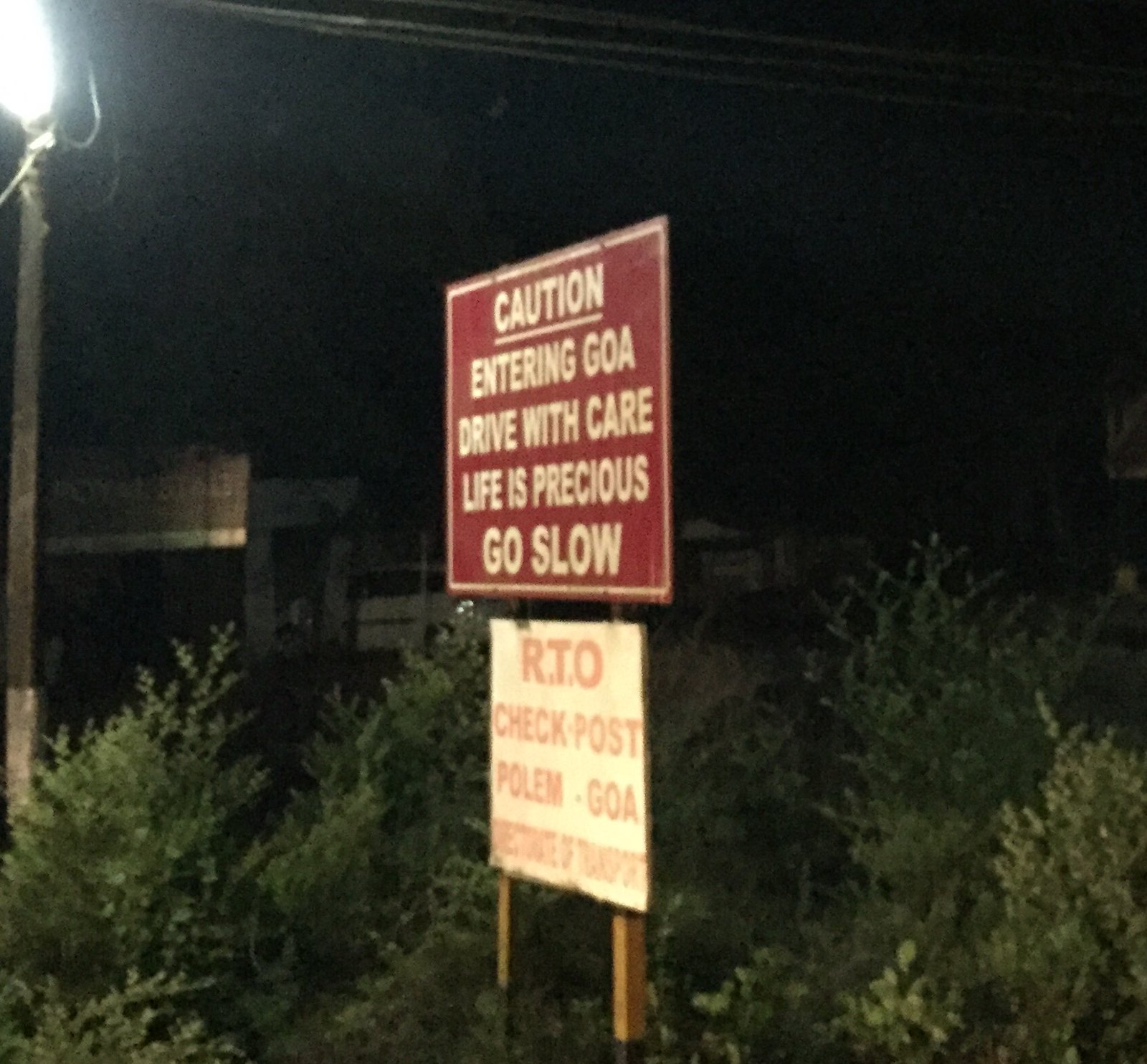This nighttime photograph captures a pair of road signs mounted on two wooden posts, anchored in a patch of small green shrubs. The top sign, red with a white border and white lettering, warns: "CAUTION! ENTERING GOA. DRIVE WITH CARE. LIFE IS PRECIOUS. GO SLOW." Directly below it, a white sign with red text reads: "RTO CHECKPOST PALM GOA," with additional, illegible text further down. The scene is framed by taller bushes in the background and illuminated by a streetlight to the left, casting a stark white light. Above, the sky is a deep black, and some indistinct buildings can be observed in the distance, contributing to the atmosphere of the scene.